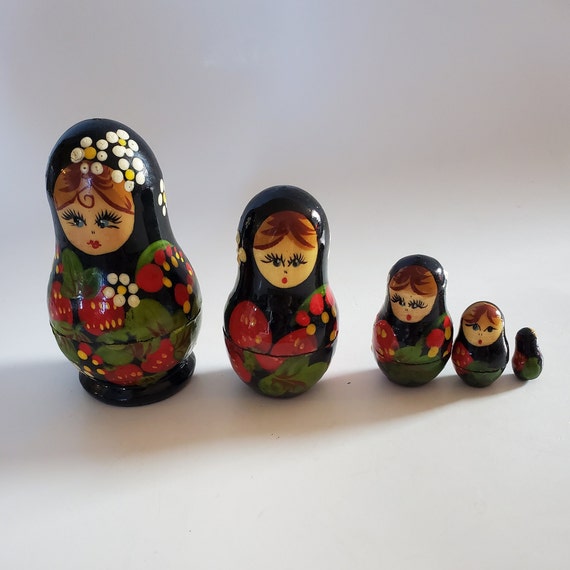This color photograph, set against a soft gray background, showcases a series of five Russian nesting dolls, or matryoshka dolls, that have been unnested and lined up progressively from largest on the left to smallest on the right. Each doll shares a similar design with variations in detailing. The largest doll, portraying a woman with brown hair and pronounced eyelashes, has decorative white and yellow flowers adorning the top of her head. Her face, adorned with large blue eyes and red lips, rests above a black base elegantly painted with clusters of strawberries featuring red berries with yellow dots and green leaves.

Moving right, the subsequent doll mirrors the largest one’s design but without the flowers on the head. Both share the same strawberry motif on a black background. The third doll, like the second, is a smaller version with identical artwork.

The fourth doll diverges slightly, presenting a baby-like face with a single strawberry painted on the black base. The smallest doll in the series appears to be a back view, showing no face but maintaining the characteristic brown hair.

Each doll, described as peanut-shaped with a base, follows the traditional nesting concept where the smaller ones fit inside the larger ones, collectively forming a family hierarchy from mother to child.